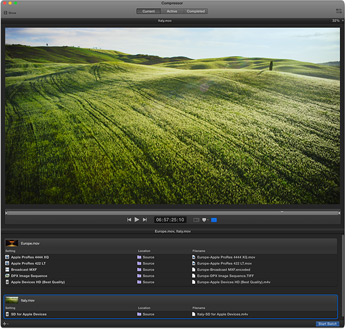A detailed screenshot, likely from a tablet or computer game, is displayed. The image has a square format and is framed by a gray border on all four sides, which is further outlined by an inner black border. At the top left corner of the screen, three small circles positioned horizontally represent the standard window control buttons in red, yellow, and green colors.

Centered within the gray border, the focus of the image is a monitor screen displaying a vibrant landscape. The display shows a neatly trimmed grassy area dotted with gentle hills, set under a pleasantly blue sky with a few scattered clouds. A solitary small tree stands towards the right side of the scene.

Directly below the monitor, in the gray border area, are control buttons. On the left side, there are play, fast forward, and rewind buttons, indicating possible media control functions. The center features what appears to be a timer or clock settings, flanked by three additional, unidentified buttons on the right. The right side of the screen displays a blurry vertical element, which seems to be up and down arrows, though the detail is not clear.

Accompanying the image, various sections of text run down the left, center, and right sides of the monitor, though the text is too small to be legible.